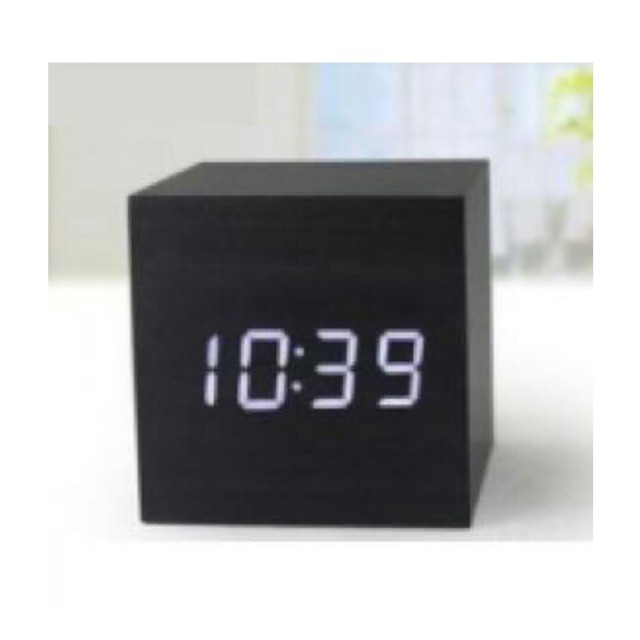This photograph captures a small, black, cube-shaped clock displaying the time 10:39. The clock's face is darker, offering a stark contrast to the white, illuminated numbers that are prominently centered. The top and sides of the clock are slightly lighter, adding dimension. It is stationed on a clean, white surface. The background is deliberately blurred, featuring soft hues of gray, green, and blue, directing full attention to the clock. The overall lighting suggests a calm, ambient atmosphere.